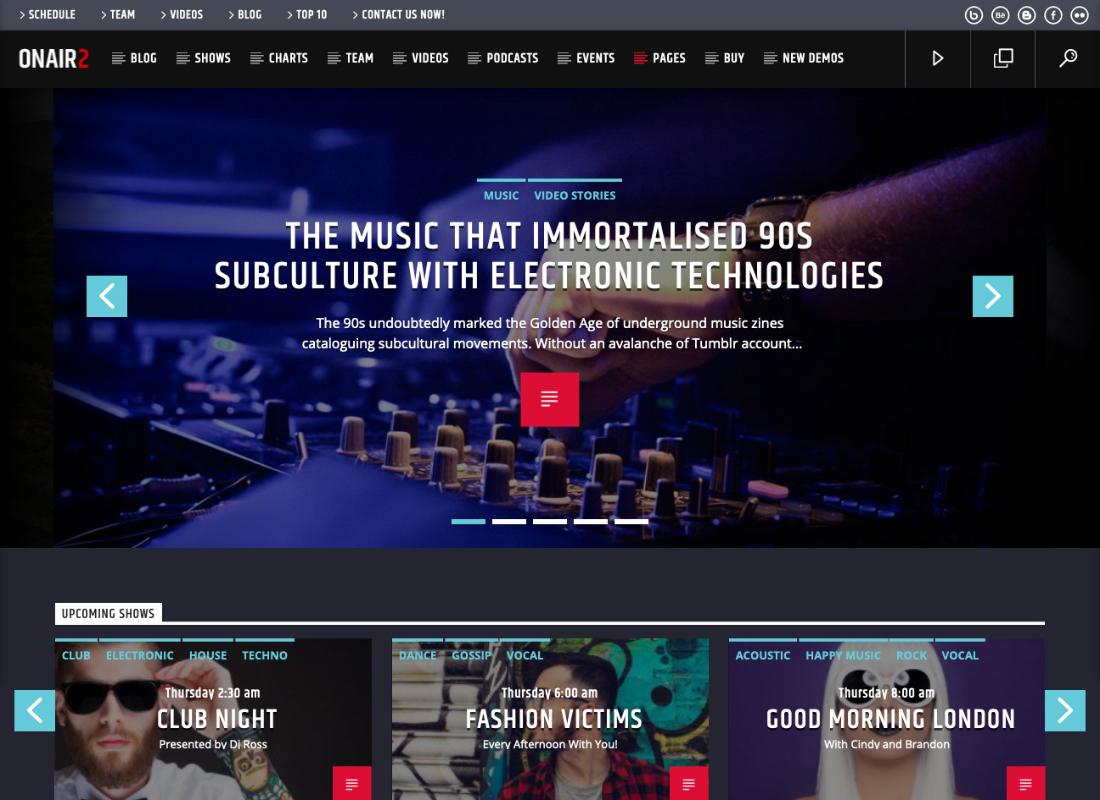This image showcases a detailed webpage layout, likely named "OnAir2." At the top, a grey navigation bar features white text with options: "Schedule," "Team," "Videos," "Blog," "Top Ten," and "Contact Us Now." To the right of these options are social media buttons.

Beneath the navigation bar, the "OnAir2" logo appears with "OnAir" in white text and "2" in red text. Adjacent to the logo, there are more menu items: "Blog," "Shows," "Charts," "Team," "Videos," "Podcasts," "Events," "Pages," "Buy," and "New Demos." Additionally, there are icons for page navigation, including an arrow, a pages logo, and a search function.

The main section of the page features an image of an individual operating music equipment. Overlaying this image is white text that reads: "The music that immortalized 90s subculture with electronic technologies. The 90s undoubtedly marked the golden age of underground music zines, cataloging subcultural movements without an avalanche of Tumblr accounts." Below this text lies a noticeable red button.

At the bottom of the webpage, there are three images, each displaying a different person. The leftmost image is captioned "Club Night," the middle image is labeled "Passion Victims," and the rightmost image is titled "Good Morning London."